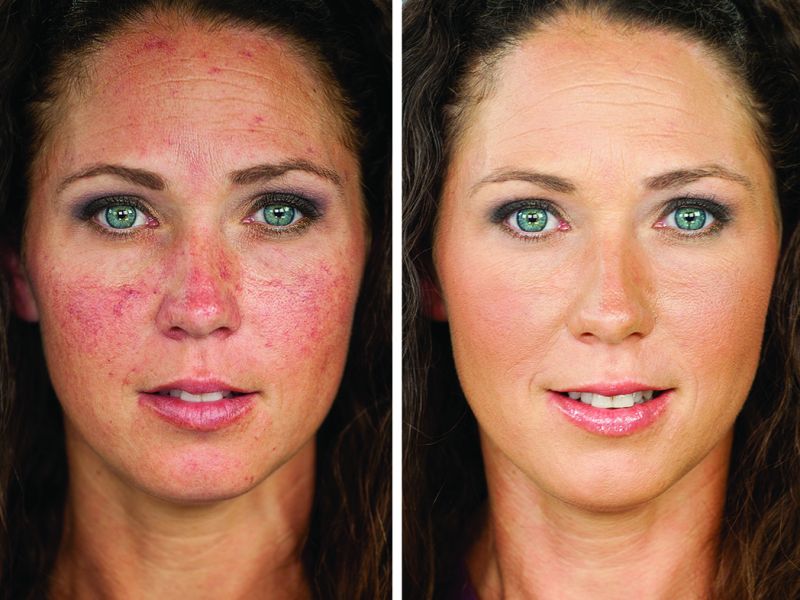This image features two side-by-side portrait-style close-up photographs of the same Caucasian woman, likely in her mid-30s to early 40s. She has bright green eyes, long brown hair that extends past the bottom of the frame, and brown eyebrows. The photos are cropped at her neck and upper forehead. In both images, she is smiling, displaying her white teeth.

In the left-hand "before" image, the woman's complexion is affected by a significant red mottled rash with acne, visible across her forehead, upper cheeks, nose, and chin. Additionally, she exhibits mild wrinkles on her forehead.

The right-hand "after" image shows the same woman with a clear, smooth, and clean complexion, suggesting the application of makeup. Her skin appears blemish-free and slightly blushed, complementing her makeup which includes a nice shade of pink lip gloss. The overall appearance is enhanced, giving her a more pleasant and refined look.